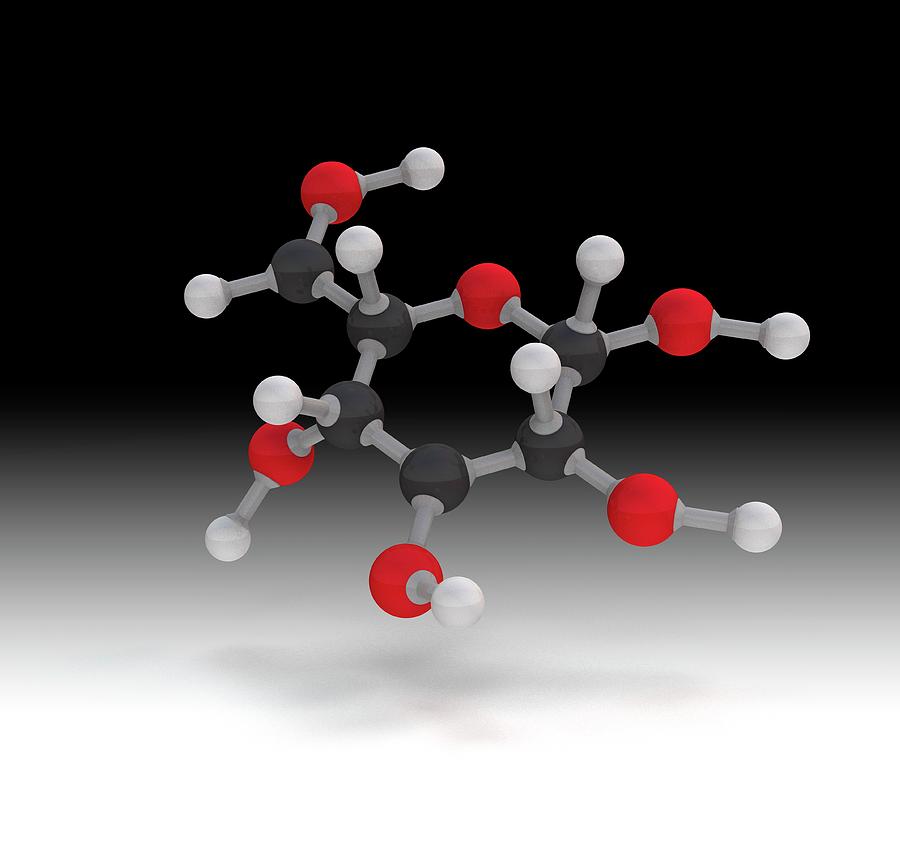The image depicts a detailed and artistic representation of a molecular structure, possibly a common molecule like water or a segment of a DNA strand, suspended in a dark background. The molecule consists of interconnected spherical "balls" attached via "rods." These balls are distinctly colored: white, red, and gray/black. The gray and red spheres are prominently similar in size, while the white spheres are notably smaller. The gray rods form a chain-like structure, visually linking the spheres. The image also captures the shadow of the molecule beneath it, adding to the three-dimensional effect. Overall, this visual representation aims to illustrate the intricate connections among atoms within a molecule, showcasing a complex yet orderly design that is commonly seen in educational science materials.